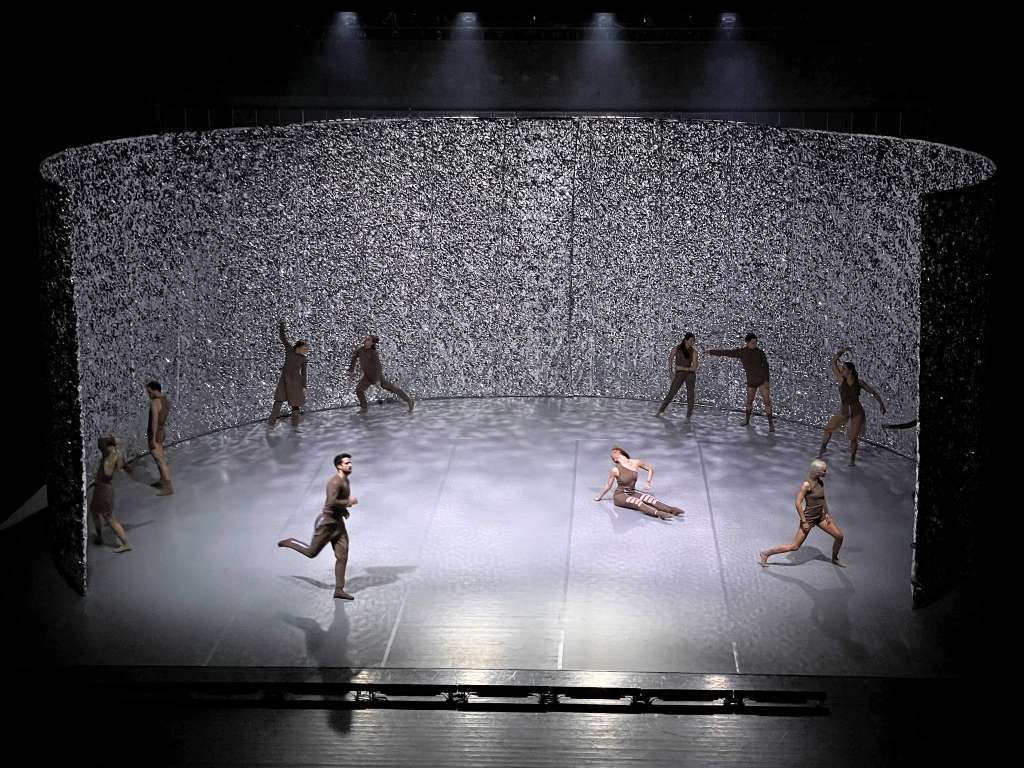In this photograph, a modern dance performance is captured from a high vantage point, possibly a balcony. The stage is surrounded by a backdrop of crinkled silver material that resembles crumpled foil, creating a striking, reflective environment. The floor shares this silver-gray hue, enhancing the cohesive visual aesthetics of the set. 

Onstage, ten dancers are enmeshed in a dynamic composition of movement, each in mid-performance. Their attire varies in shades of brown, with some sporting sleeveless tops, others in pants, and still others in dresses, giving a diverse yet uniform look. The first dancer on the left, a man, appears to be running, his right leg lifted. To his left, another performer, likely a woman, faces the crinkled silver wall. Next, a man in shorts also turns toward the wall. 

Another dancer, with long sleeves and pants, stands center stage with an arm raised, seemingly engaged in an introspective moment. Adjacent to them, another performer extends their left leg and looks skyward, embodying the fluidity of the performance. 

Towards the right of the stage, one dancer points their toe elegantly while gazing at a nearby partner, who reciprocates with an outstretched arm, wearing shorts. Nearby, a dancer strikes a ballet-like pose with her right arm elevated and toe pointed. Completing the scene, a solitary arm emerges from the group, hinting at yet another dancer in motion.

On the bottom right, a woman poses with her knee bent and right leg extended, facing the wall, while another dancer toward the center of the stage leans back gracefully over her right shoulder, dressed in an asymmetrical one-shoulder top and pants. This rich tableau of movement and expression captures the essence of the choreographed performance, set against a shimmering, unconventional backdrop.